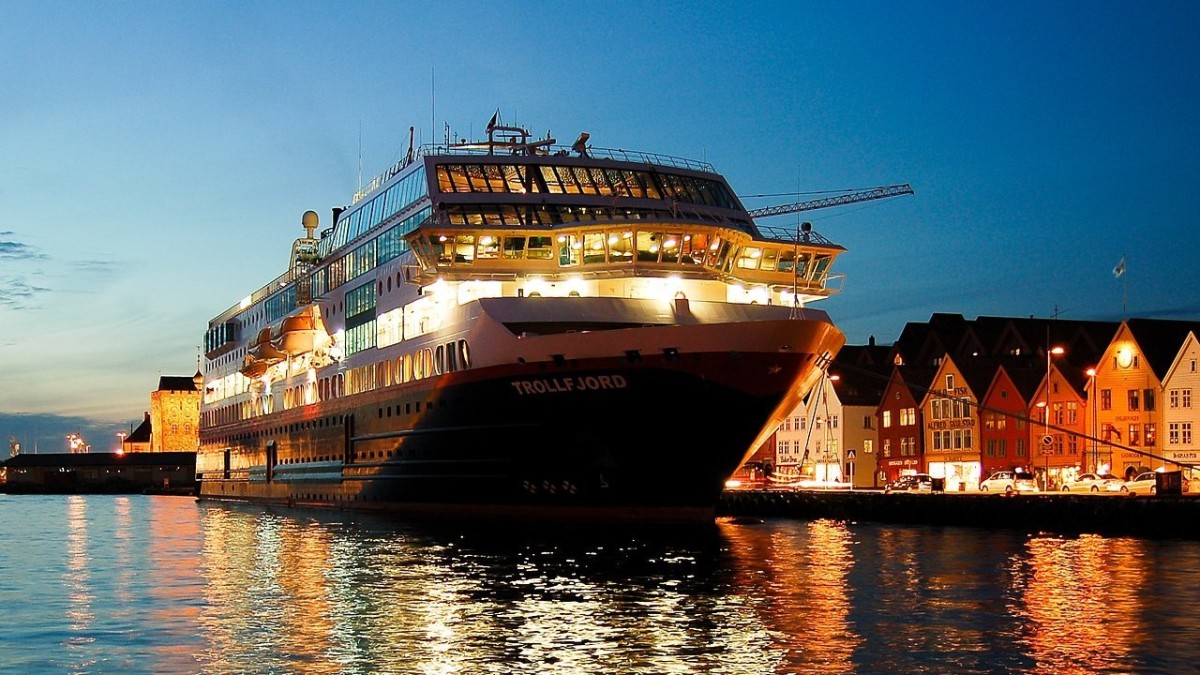This photograph captures an evocative scene taken outdoors during dusk, with a deepening blue sky that transitions from lighter hues on the left to darker shades on the right as night approaches. Dominating the scene is a large luxury cruise ship named "Trollfjord," clearly visible through its brightly illuminated windows and multiple stories. The vessel's design features a black lower hull, a red stripe, and a white section, culminating in an overall dark gray body with "Trollfjord" inscribed in white text on the side. The ship, which possibly has amenities such as dining spaces and guest rooms, is reflecting its vibrant lights on the water below. Positioned near a tranquil shoreline, the background reveals a waterfront town with a series of houses, streetlights, and additional reflections cast upon the water. Contrasting the ship’s grandeur, the houses have flat-faced, pointed rooftops, and a variety of colors. Adding to the industrial feel, a crane is seen extending from the boat, subtly integrating into the serene landscape.